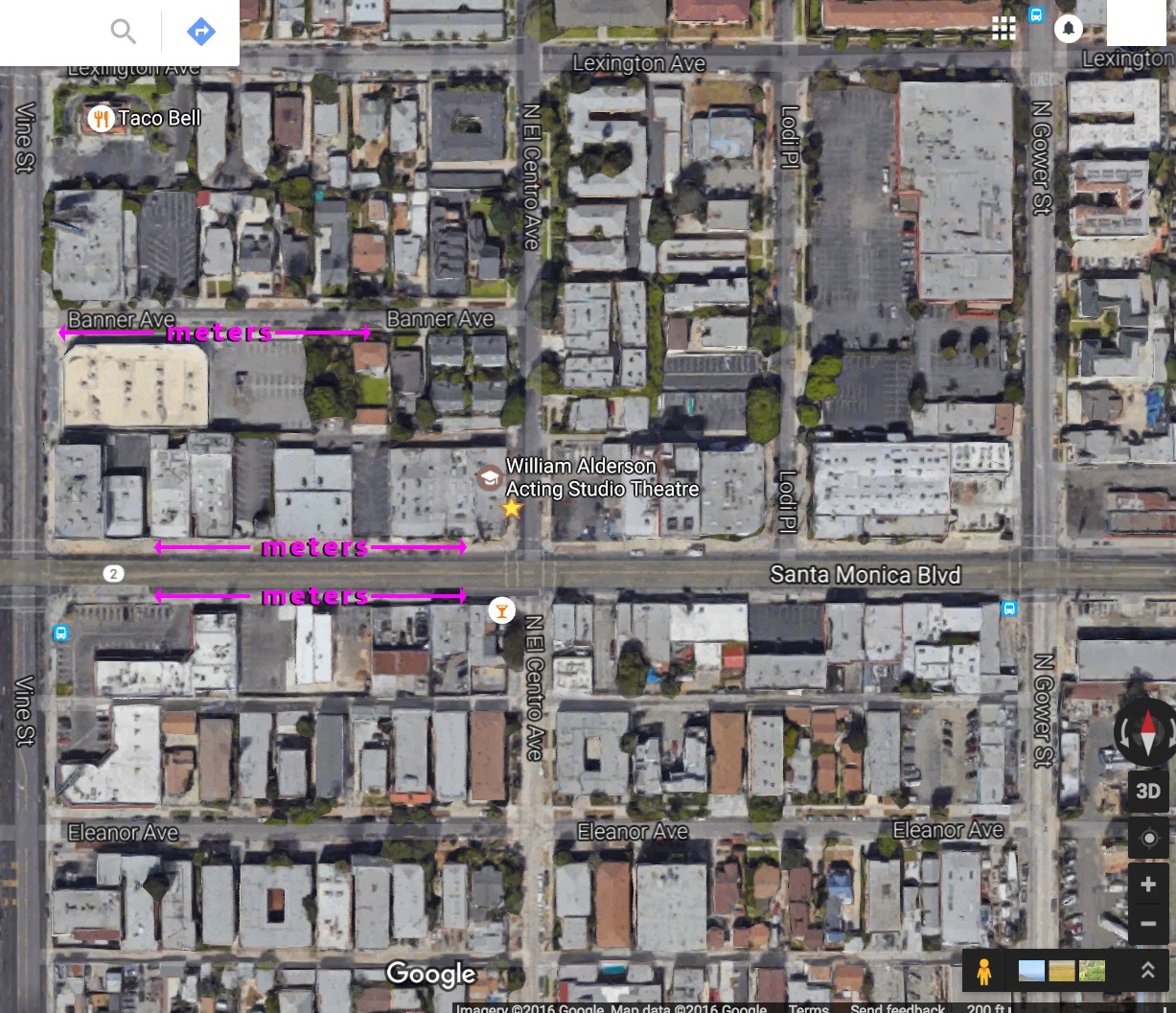A detailed aerial view of a neighborhood is depicted in this Google Maps image, showcasing various streets and landmarks. The central streets visible include Main Street and Banner Avenue. The William Alderson Acting Studio is marked, alongside meters highlighted in purple text. Prominent roads such as Lexington Avenue and Santa Monica Boulevard are also visible. 

The rooftops, primarily in shades of gray and brown with a few black and white ones, create a patchwork across the scene. At the bottom of the image, the word "Google" is displayed, with a 3D label in white print, signifying the three-dimensional perspective of the map. Three tiny inset images and a small yellow Street View icon are positioned to the side, providing additional navigation options. A magnifying glass icon at the top suggests the presence of a search feature. Notably, the image also identifies a Taco Bell and Eleanor Avenue, adding more context to the neighborhood layout.